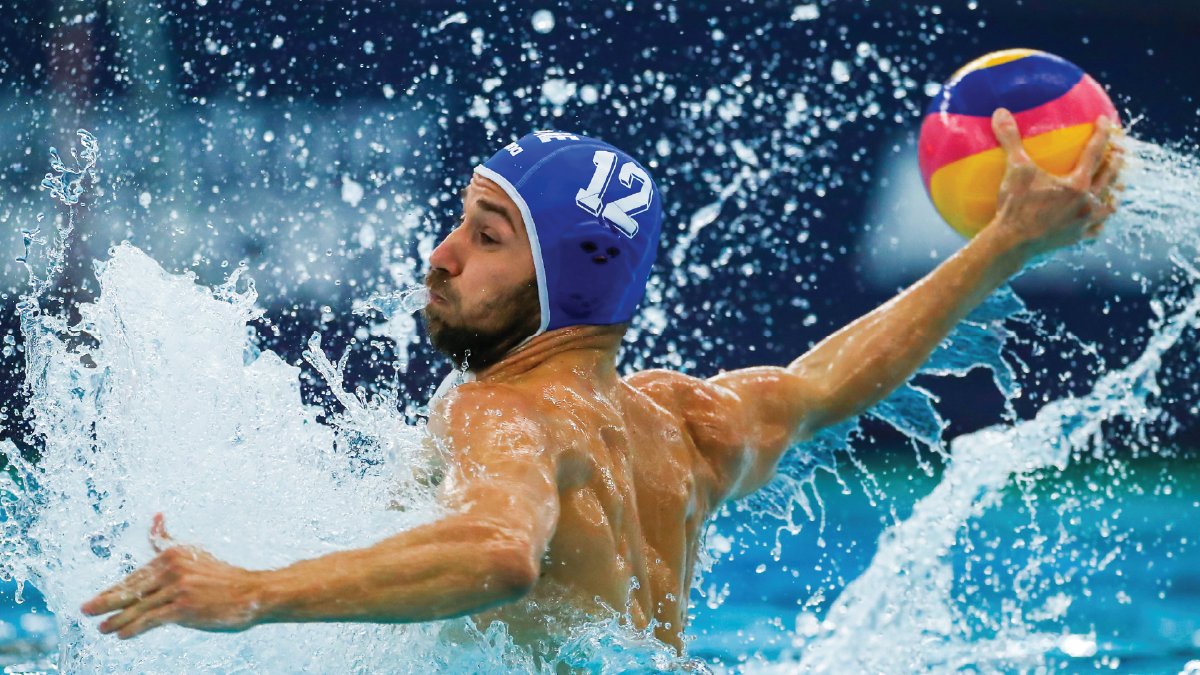This is a highly detailed action photograph of a water polo player, captured mid-motion with remarkable clarity. The athlete is a muscular, white male with a brownish-black beard, wearing a blue cap marked with the number 12 in white. He is shirtless and in the midst of a powerful movement, winding up to throw a multicolored ball that features shades of pink, blue, and yellow. His right arm is stretched way back, gripping the ball tightly in preparation for an intense throw, while his left arm is extended forward to support his targeting. The expression on his face is one of sheer determination. The image captures a dramatic splash around him, with water droplets and waves suspended in midair, highlighting the explosive energy of the moment.